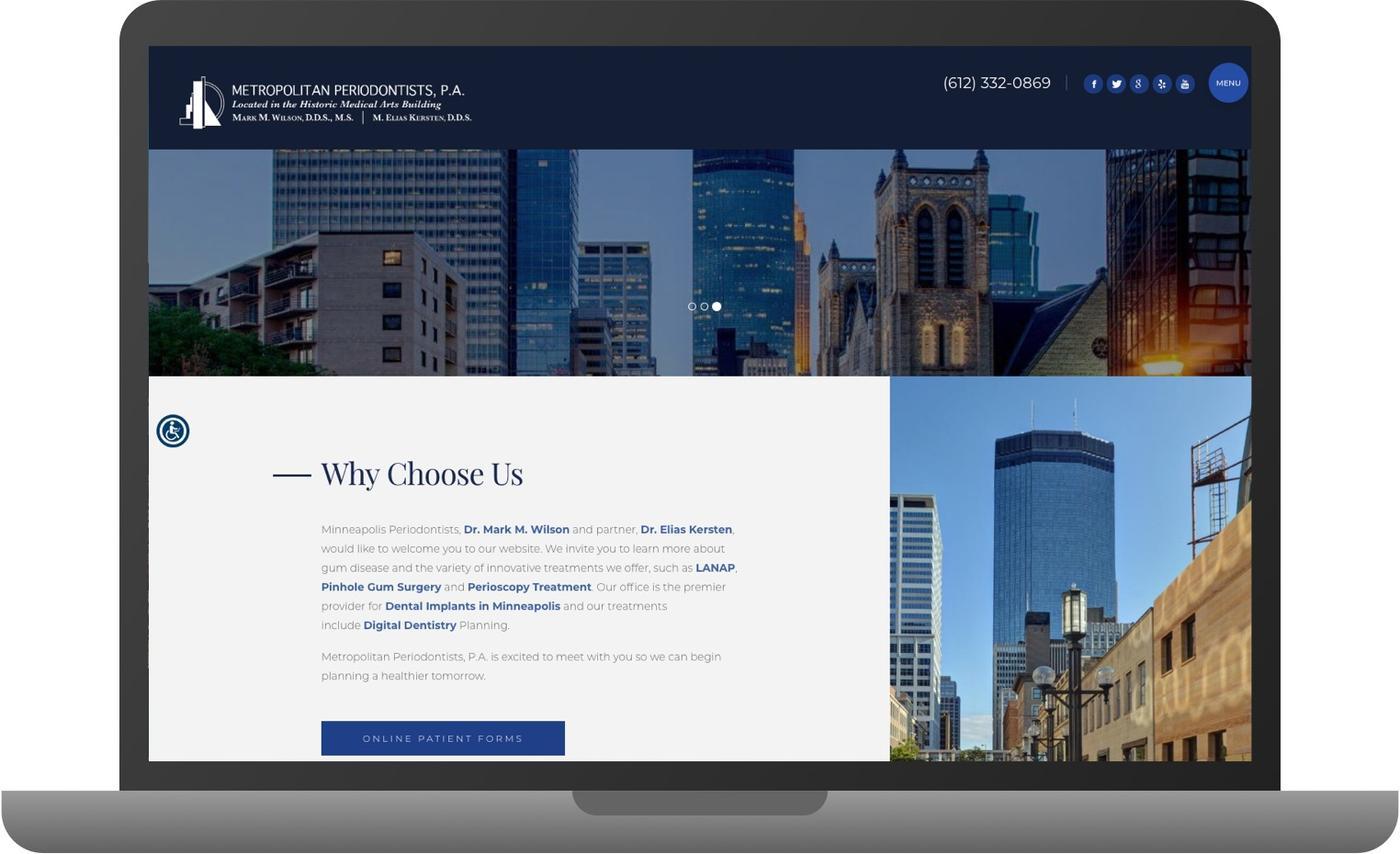The image showcases a web page displayed on a superimposed, centrally positioned laptop screen. The screen layout is predominantly rectangular, much wider than it is tall, and features a horizontal blue border at the top. Within this blue border is the white-font text "Metropolitan Percussionist PA" alongside a building logo. To the right, there's a phone number in white, accompanied by blue circular icons with white symbols indicating links to various social media platforms.

Beneath the header, there is a striking cityscape image displaying several tall, glass-clad buildings. Following this, another horizontal divider spans across the screen. Below this divider, a white box contains the text "Why Choose Us" in black, with additional descriptive text and blue hyperlinks underneath. Towards the bottom is a long, narrow blue rectangular box containing the white-font text "Online Patient Forms."

To the right is a vertically or portrait-oriented cityscape image featuring a tall, octagonal-shaped glass building in the background. Adjacent to it on the left is another tall building, while several shorter structures made of steel, brick, or stone can be seen in the foreground on the right.